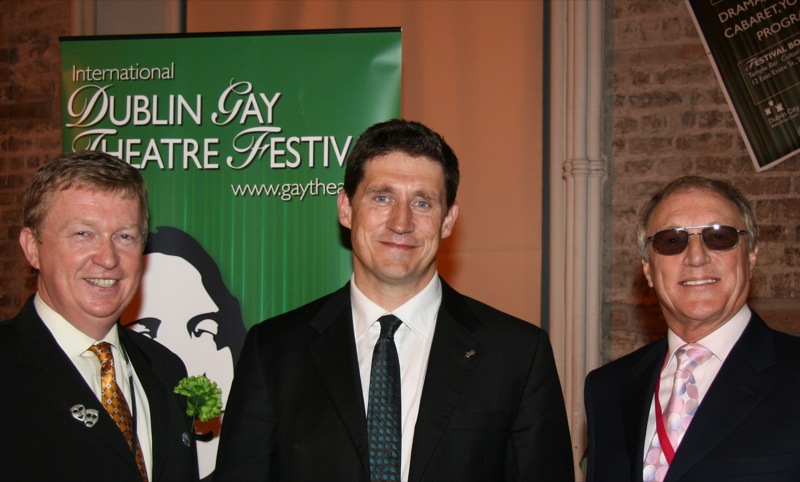This indoor photograph captures three men, each dressed in dark suits with white undershirts and unique ties. The man in the center wears a blueish-green tie with a dot pattern and stares directly at the camera. To his right, a man with a white tie adorned with silver or off-pink polka dots and wearing sunglasses also looks straight ahead; he sports a distinctive red sash across his chest. On the left stands a man with a golden tie featuring a diamond pattern and a pin of a comedy and tragedy mask, smiling at the camera. All three appear to be in their 50s or 60s and share dark hair. They stand against a backdrop of a green banner that reads "International Dublin Gay Theatre Festival" along with a partially visible URL. The brick walls to either side of the banner accentuate the indoor setting.